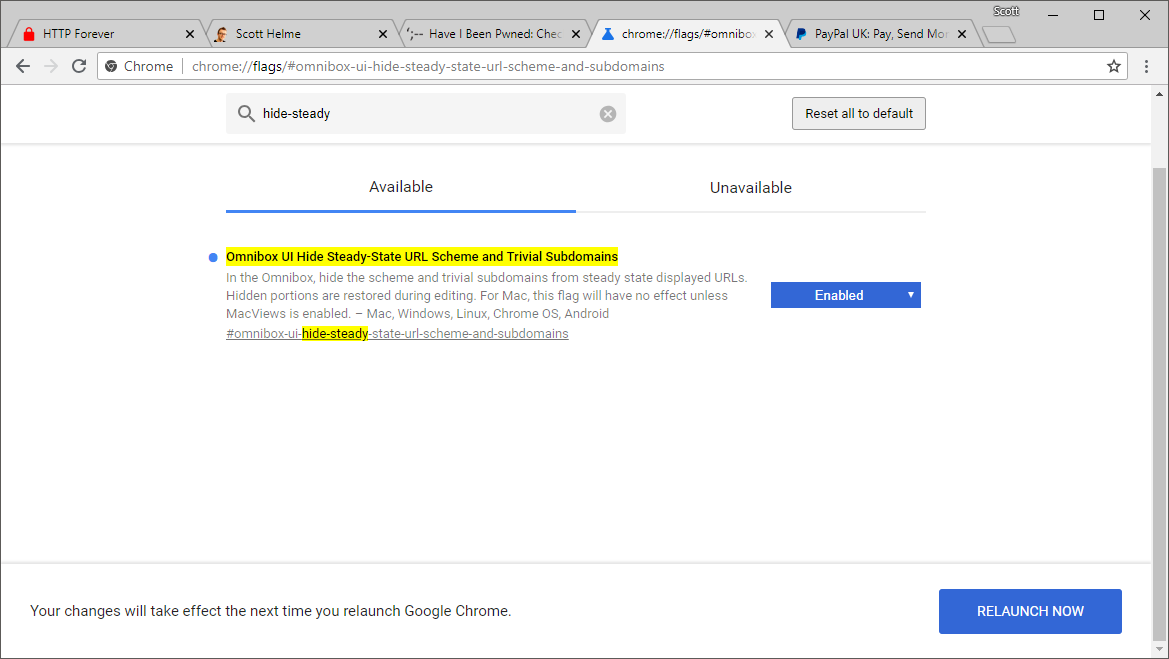The image showcases a computer monitor displaying the Google Chrome browser with five open tabs: "HTTP Forever," "Scott Helm," "Have I Been PWNED," "PayPal," and "UK Pay." The current tab being viewed is the "Chrome flags" page, accessible via the URL "chrome://flags."

In the browser's address bar, one can see the navigation arrows (left and right), a refresh button, and the URL "chrome://flags." Below the address bar is a search box, which has a magnifying glass icon and the placeholder text "Hide steady." To the right of this search box is a button labeled "Reset all to default."

The page itself is divided into two sections: "Available" and "Unavailable," with the user currently viewing the "Available" section. Prominently highlighted in yellow is a feature titled "Omnibox UI Hide Steady-State URL Scheme and Trivial Subdomains." The description below explains that this feature hides the scheme and trivial subdomains from steady-state displayed URLs in the Omnibox, making them visible again during editing. It mentions that this feature affects various platforms including Mac, Windows, Linux, Chrome OS, and Android, but notes that it has no effect on Mac unless "Mac Views" is enabled. The feature is tagged with "Omnibox UI Hide Steady-State URL Scheme and Subdomains" as a hashtag.

To the right of the highlighted description is a blue "Enable" button for activating this feature. Further down, there is a message stating that "Your changes will take effect the next time you relaunch Google Chrome," accompanied by another blue button labeled "Relaunch now."